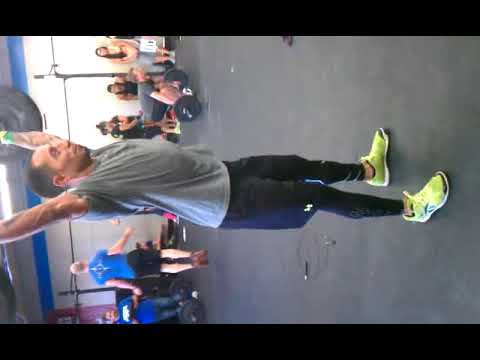The photograph, oriented sideways, captures a man weightlifting, positioned centrally with his arms extended above his head, gripping a barbell loaded with weights. He is a short-haired Caucasian man with a slight beard, wearing a gray t-shirt and black shorts featuring a white Under Armour emblem near the knee. His outfit includes light green shoes with black toes and white accents, complementing his tight black ankle socks. The man stands on a flat dark gray surface, exuding a sense of focus and effort.

In the background, several people are visible along the wall, with two dressed in black, one in a yellow shirt, and another engaged in jumping rope with a blue shirt, black shorts, and brown shoes. Additionally, another individual can be seen in a squatting position, preparing to lift a barbell. The upper and lower portions of the image are bordered by black rectangular strips, slightly cropping the scene. This detailed composition highlights the dynamic activity within the room and the intensity of the central figure's weightlifting moment.